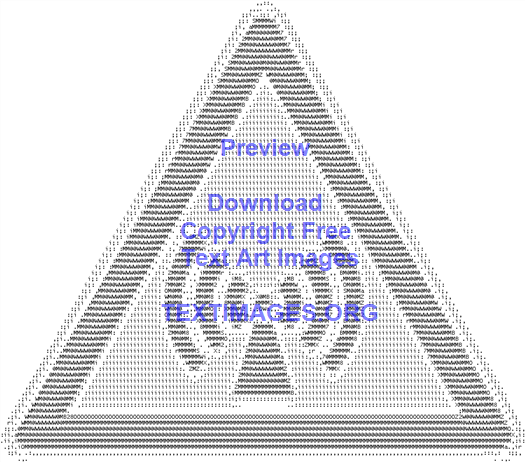This image is a square piece of text art with a crisp white background, featuring a precisely shaped equilateral triangle pointing upwards. The triangle is meticulously crafted using a spectrum of gray and black letters or dots, creating a gradient effect where the outer edges are lighter and the center progressively darkens. Nestled within this composition is a series of concentric triangles: a dark-bordered middle triangle and a lighter inner triangle that houses an illustration resembling a lighthouse or broadcasting tower emitting sound waves. Overlaying the entire visual in transparent purple or blue font is the text: "Preview Download Copyright-Free Text Art Images TextImages.org."